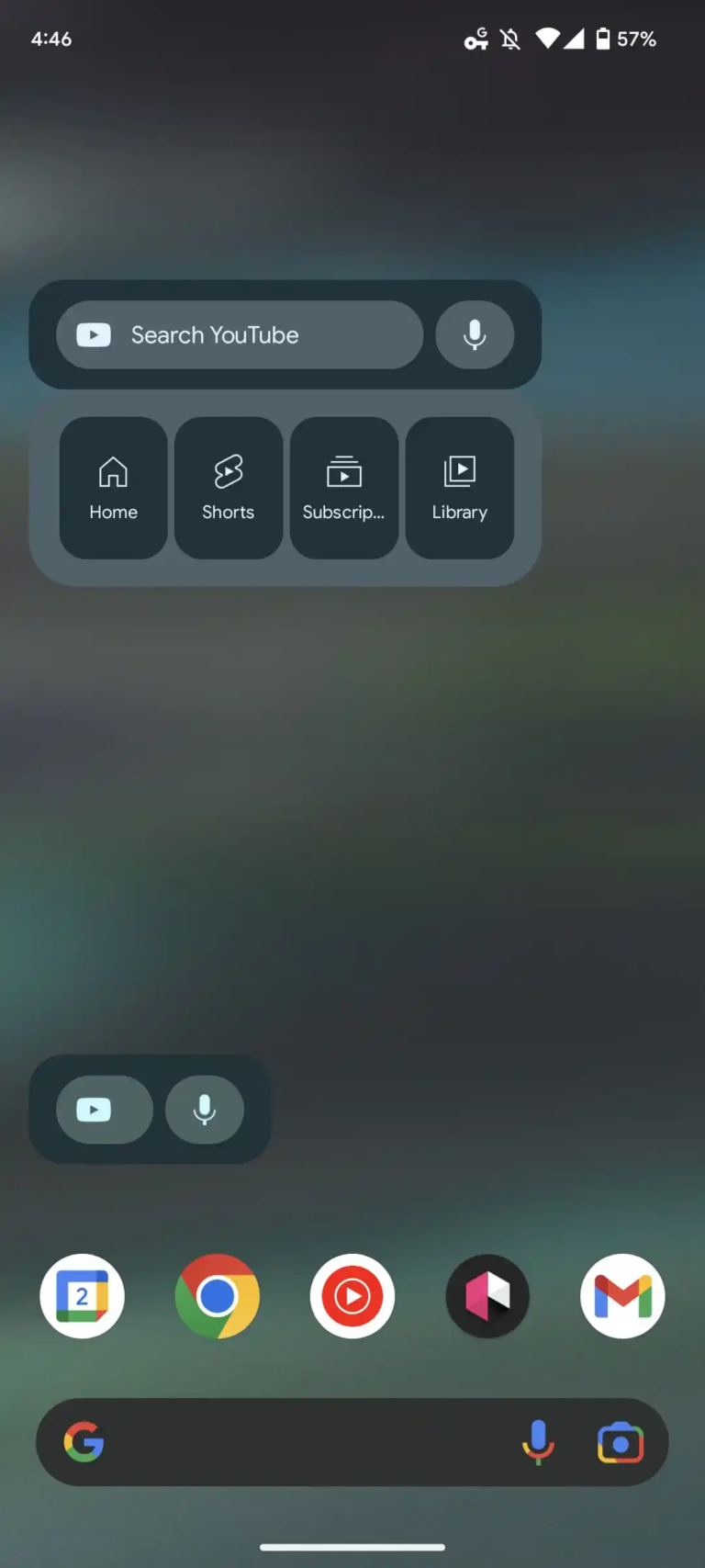This image appears to be a screenshot from a smartphone display, taken at 4:46 with the battery at 57%. Along the top bar, several icons indicating connectivity and notifications are present. Below this, there is a prominent YouTube search area flanked by a search bar and a microphone icon.

Further down, within a green, rounded rectangular section, lie four essential navigation buttons for YouTube. Each button has a black icon with descriptive text below:

- "Home" accompanied by a house icon.
- "Shorts" displaying a rotated 'S.'
- "Subscriptions," presented with a play button inside a box.
- "Library," again showing a play button within a box.

The background of the screen has a blurred, green and blue camouflage-like appearance. Near the bottom of the screen, a clickable play button and a microphone icon are visible. At the very bottom rests a Google search box that includes a microphone and camera input options.

Spread across the middle section are five app icons: one showing the number ‘2,’ Google Chrome, YouTube, Google Mail, and another unidentified icon.